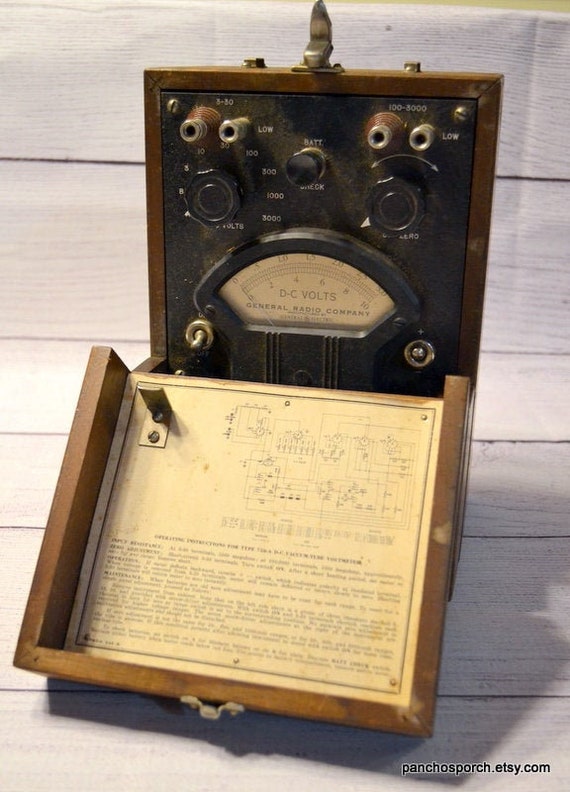This photo showcases a vintage electronic device, likely from the 1920s or 1930s, produced by the General Radio Company. It's housed in a wooden case with a lid that features a detailed schematic diagram of the device's electrical flow and an unreadable paragraph of instructions. The device itself is the focal point, equipped with a DC voltmeter, several dials, and switches likely used to adjust voltage. There are four distinct plugs visible, underscoring its multifunctionality. The background is a simple white-painted wooden surface. Notably, there is a clasp on the case for securing it shut, and a stamp at the bottom indicates it is being sold on PanchoSports.etsy.com.